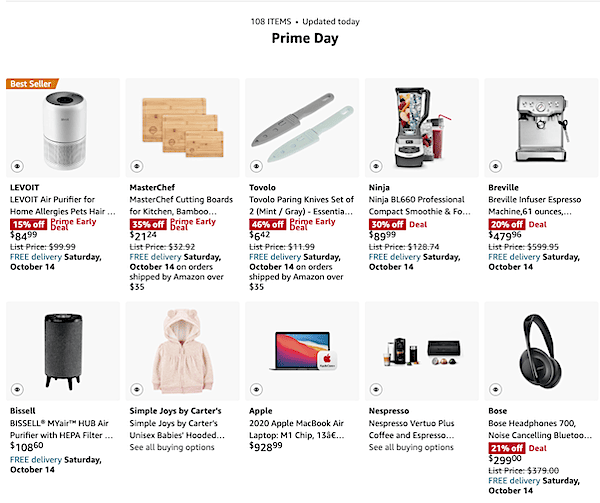The image features a neatly arranged display of ten products, organized into two rows of five blocks each. Each block showcases a different product. Centered at the top of the image, there's a label that reads "108 items. Updated today" in a clear and understated font. Directly below this, the text "Prime Day" stands out prominently in a larger, bold black font.

In the first row, from left to right:
1. An air purifier for home allergies and pet hair, priced at $84.99.
2. A MasterChef cutting board, priced at $21.24.
3. A knife set including paring knives, priced at $6.42.
4. A Ninja compact blender, priced at $18.99.
5. An espresso machine, priced at $479.96.

In the second row, the first item is:
1. Another air purifier, priced at $108.60.

The visual organization and pricing of the items emphasize the variety of products available on this Prime Day promotion.